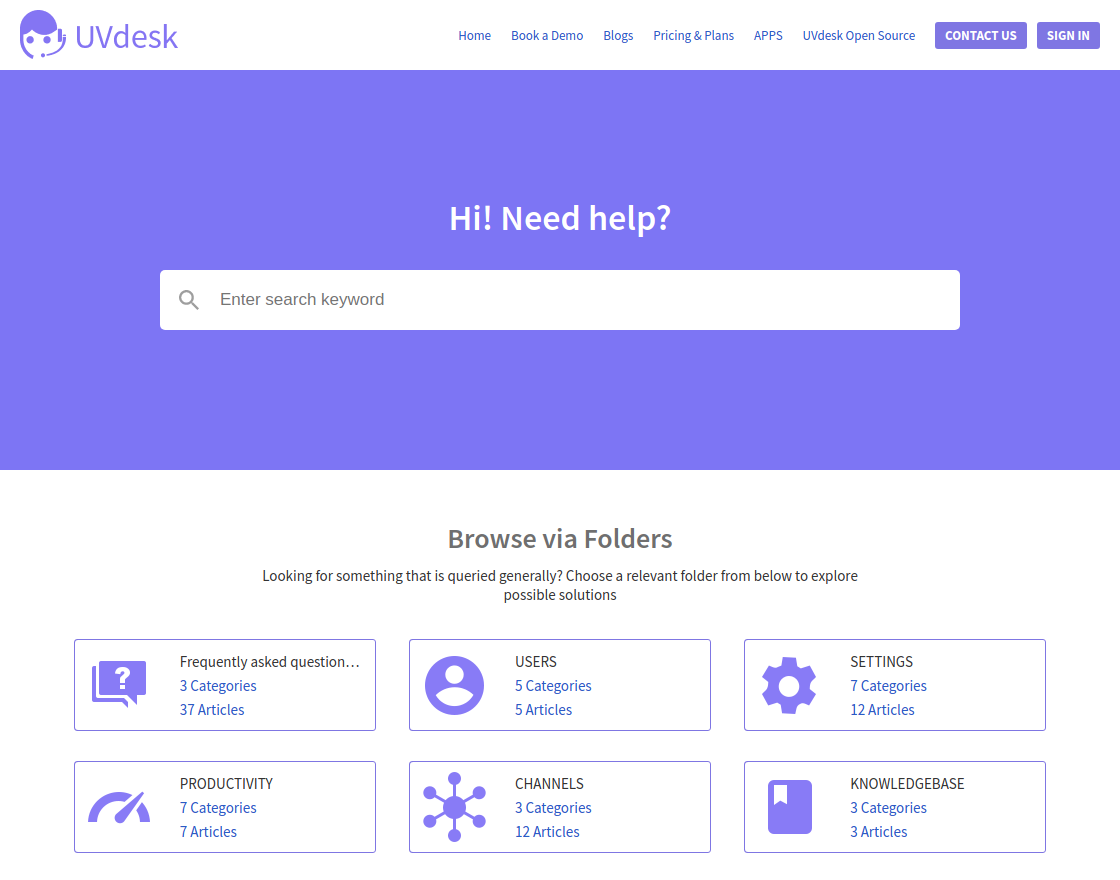This screenshot depicts a webpage with a predominantly white background. At the very top, there is a purple silhouette of a person's head wearing a headset. The image shows the person without a mouth, with the headset's microphone positioned near the left ear.

Next to the silhouette, "UV" is written in thin uppercase purple letters, followed by "desk" in lowercase purple letters. The entire header section is white. Moving to the middle of the top banner, there are navigation options written in small purple uppercase letters: "HOME," "BOOK A DEMO," "BLOGS," "PRICING," "PLANNING," and "APPS." Additionally, the phrase "UVdesk" is presented with "UV" in uppercase and "desk" in lowercase in purple font, accompanied by the term "Open-source."

Located on the right side of the top banner are two small dark purple boxes spaced apart, labeled "Contact Us" and "Sign In" in small white letters.

Directly beneath the top section, there is a large light purple rectangular banner extending almost to the middle of the page. This banner features a search box with the text "Hi! Need Help?" in white font. The search box itself contains a diagonal magnifying glass icon along with the prompt "Enter search keyword."

Further down, the page retains its white background, and a dark gray font introduces the section: "Browse via Folders." Below this heading, smaller text in the same color reads: "Looking for something that is queried generally? Choose a relevant folder from below to explore possible solutions."

The content is organized into two rows of three boxes each, labeled as follows:
1. Frequently Asked Questions
2. Users
3. Settings
4. Productivity
5. Channels
6. Knowledge Base

Each box is clickable and presumably links to categories and articles relevant to these topics.

This detailed description should provide a comprehensive understanding of the visual elements and layout of the webpage screenshot.